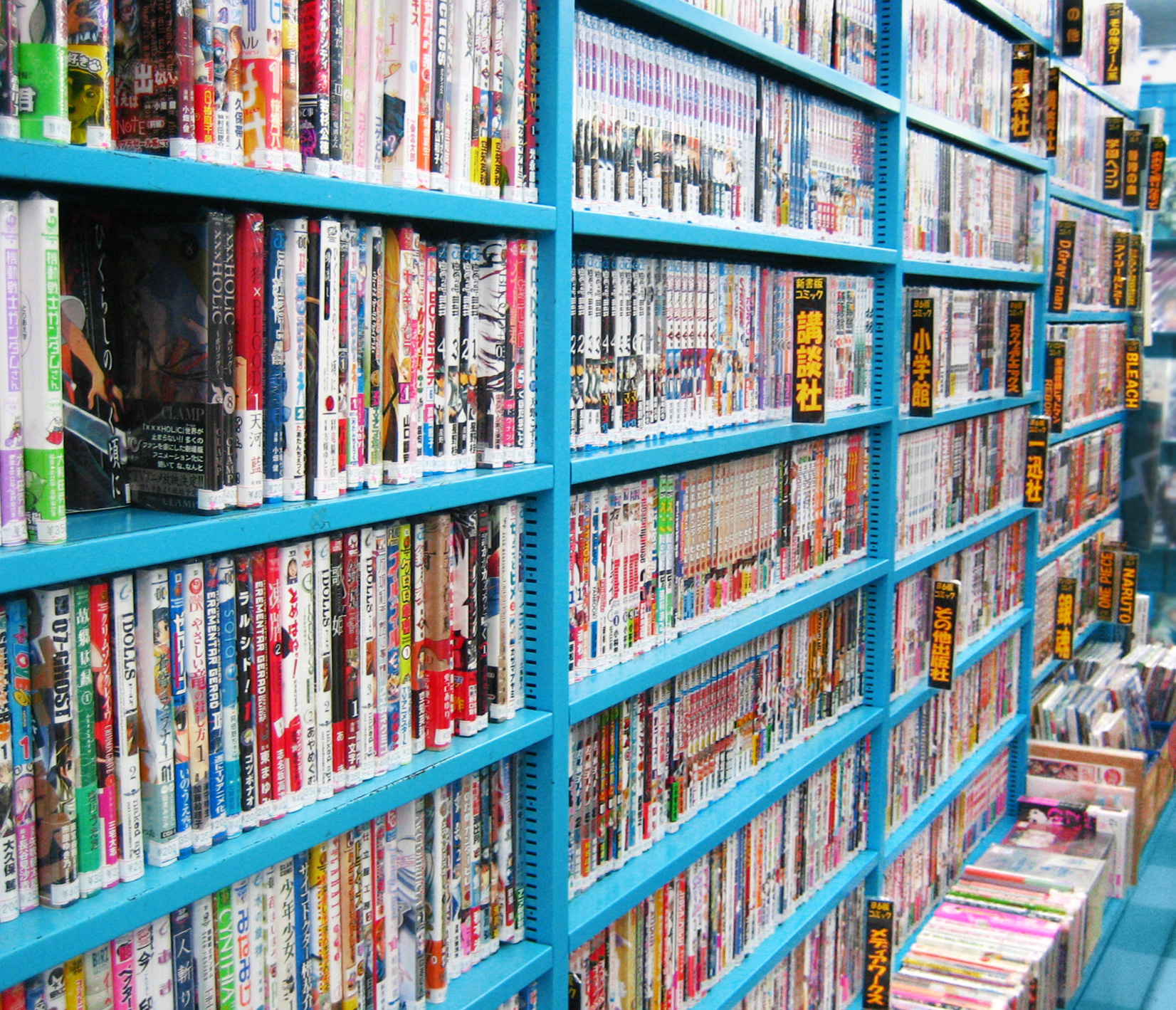The image depicts a vibrant indoor scene, likely in a Japanese bookstore or DVD shop, characterized by electric blue metal shelves loaded with DVDs. Each shelf, tightly packed with colorful DVDs, displays meticulous organization—though a few have small gaps, and some DVDs even rest on the blue-tiled floor, leaning against the shelves. Tags with black backgrounds and yellow Japanese characters jut out at random intervals, more densely scattered in the background than the foreground. The perspective of the photo runs from a close-up view on the left, receding to the right, showcasing at least four shelves teeming with potentially thousands of DVDs, suggesting a highly organized collection. The visible floor space, an amalgamation of blue tiles, further emphasizes the vibrant blue theme of this meticulously arranged shop.